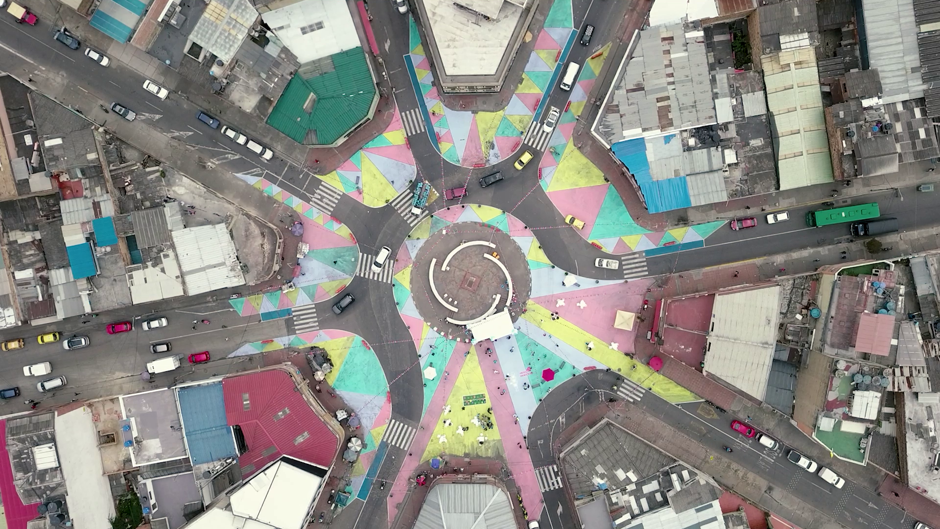This aerial photograph captures a vibrant roundabout in the heart of a city, surrounded by one-story buildings that stretch as far as the eye can see. The cityscape is adorned with a kaleidoscope of pastel colors, with the roundabout itself painted in cheerful hues of yellow, pink, green, and blue. Vehicles, including numerous brightly colored cars and green buses, are seen navigating toward and around the roundabout. The rooftops of the buildings are equally colorful, featuring shades of green, maroon, white, and blue, with some even displaying stripes. There are white structures within the city center that may be benches or installations, adding to the lively atmosphere. The photograph, likely taken from a drone or helicopter, offers a strikingly colorful and dynamic view of urban life.